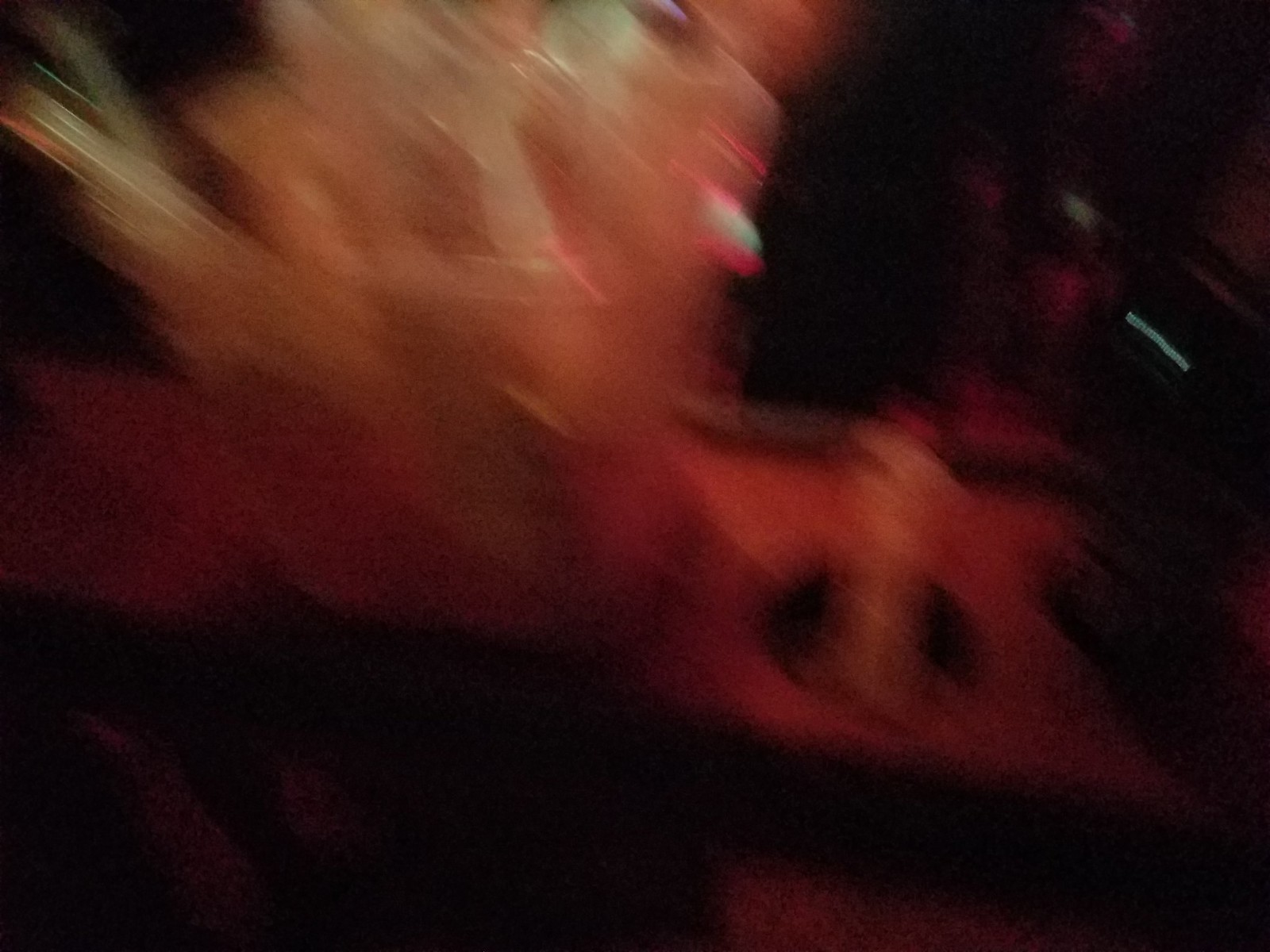This color photograph, captured with a slow shutter speed in a presumably nighttime setting, is extremely blurry, making it difficult to discern details clearly. Dominantly dark, with substantial black areas, the image appears to depict a translucent or clear, rectangular plastic box containing similarly clear or white items, positioned on a red surface. Adjacent to the box, there is a noticeable hole in the surface, from which an oval structure emerges. The scene includes a variety of elements: at the top right, a whitish object that might resemble a coffee machine, and nearby, a light blue rectangle bordered by black. The image also hints at a possible human figure dressed in white and perhaps a circular object behind them, suggesting a rapid motion that gives the scene a street-like, dynamic quality. The lower portions of the image show dark black regions interspersed with streaks of white, red, and orange, adding to the chaotic and uncertain atmosphere of the photograph.